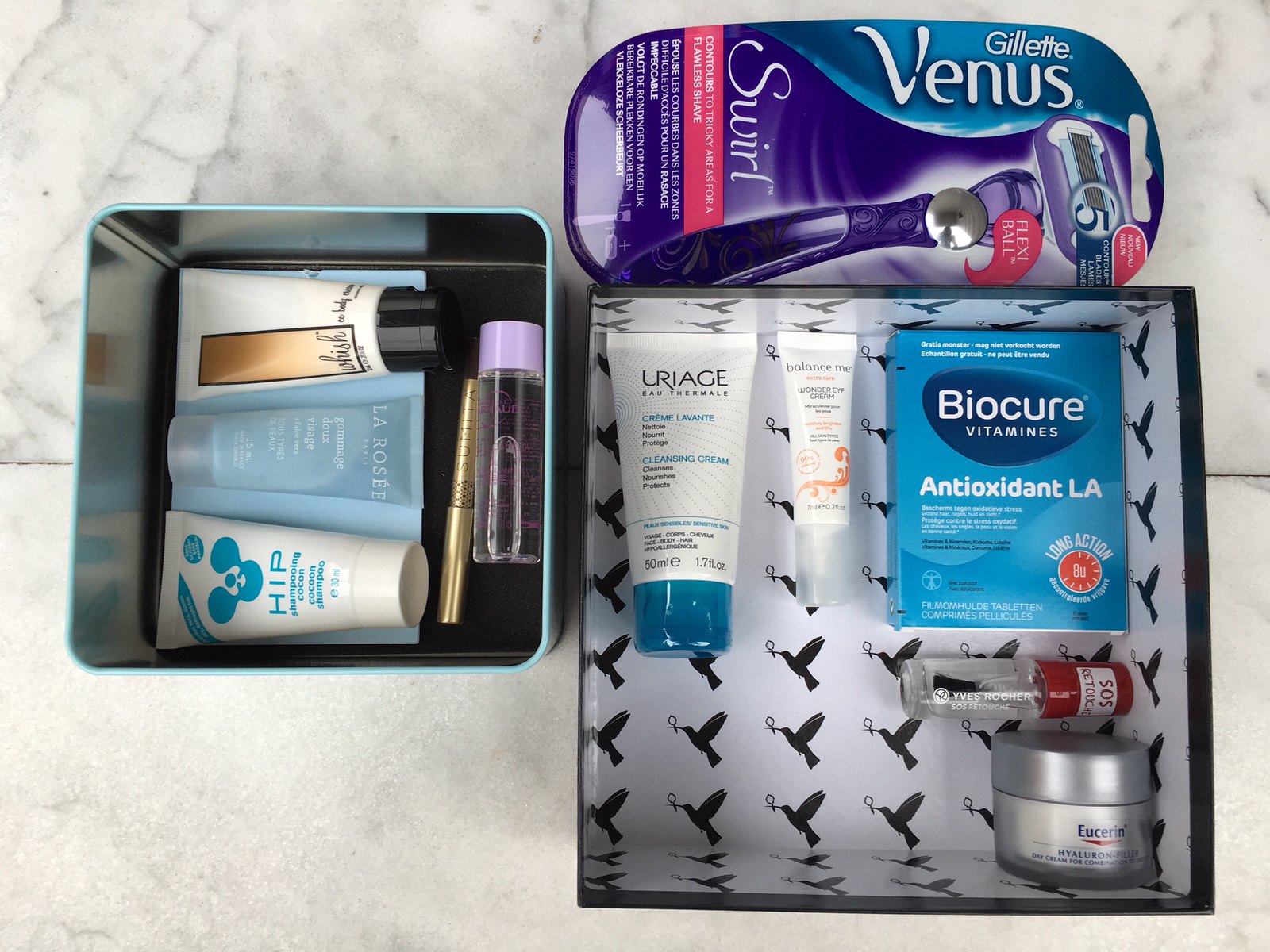This image showcases a variety of facial care products organized within two separate boxes. In the top right corner, there is a Gillette Venus razor encased in a purple box adorned with "Swirl" written on it in red stripes and accents. The box also features blue accents at the top, with "Gillette Venus" prominently displayed in white letters, indicating it's a women's razor.

To the left, there is a box containing an assortment of creams lined up in a row. The middle cream has a bluish-clear tint, labeled "La Rose." Above it, a white cream with an illegible gold square label is visible. Below, there is a white cream branded with the word "hip," featuring blue mouse ears on a white bottle. This box also contains a clear liquid in a container with a purple lid and a gold-colored pencil-like object to the right.

On the right side of the image, another box reveals its contents. In the bottom left space, there are two different creams placed on top of it. One cream is labeled "La Rage," and next to it, the other cream reads "Bio Cure Vitamins," with "Antioxidant LA" written on it. In the bottom right corner of this box, there is a Eucerin cream.